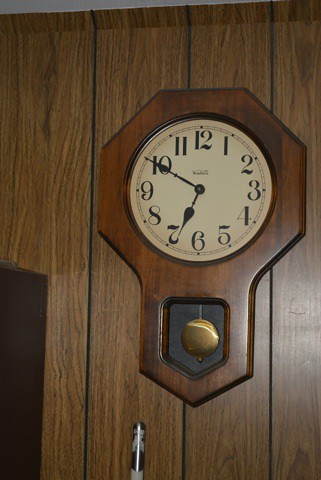The image features a classic, round-faced clock mounted on a rustic wooden wall with a rich brown hue. The clock displays the time as approximately 6:50. Surrounding the clock face are clear black numerals, arranged in standard order from 12 at the top to 11. Beneath the face, a golden pendulum can be seen, designed to swing back and forth with each hour's chime. The clock is encased in a brown wooden frame that seamlessly blends with the wooden wall. Adjacent to the clock is a noticeable brown stain, adding a touch of character to the wooden backdrop.